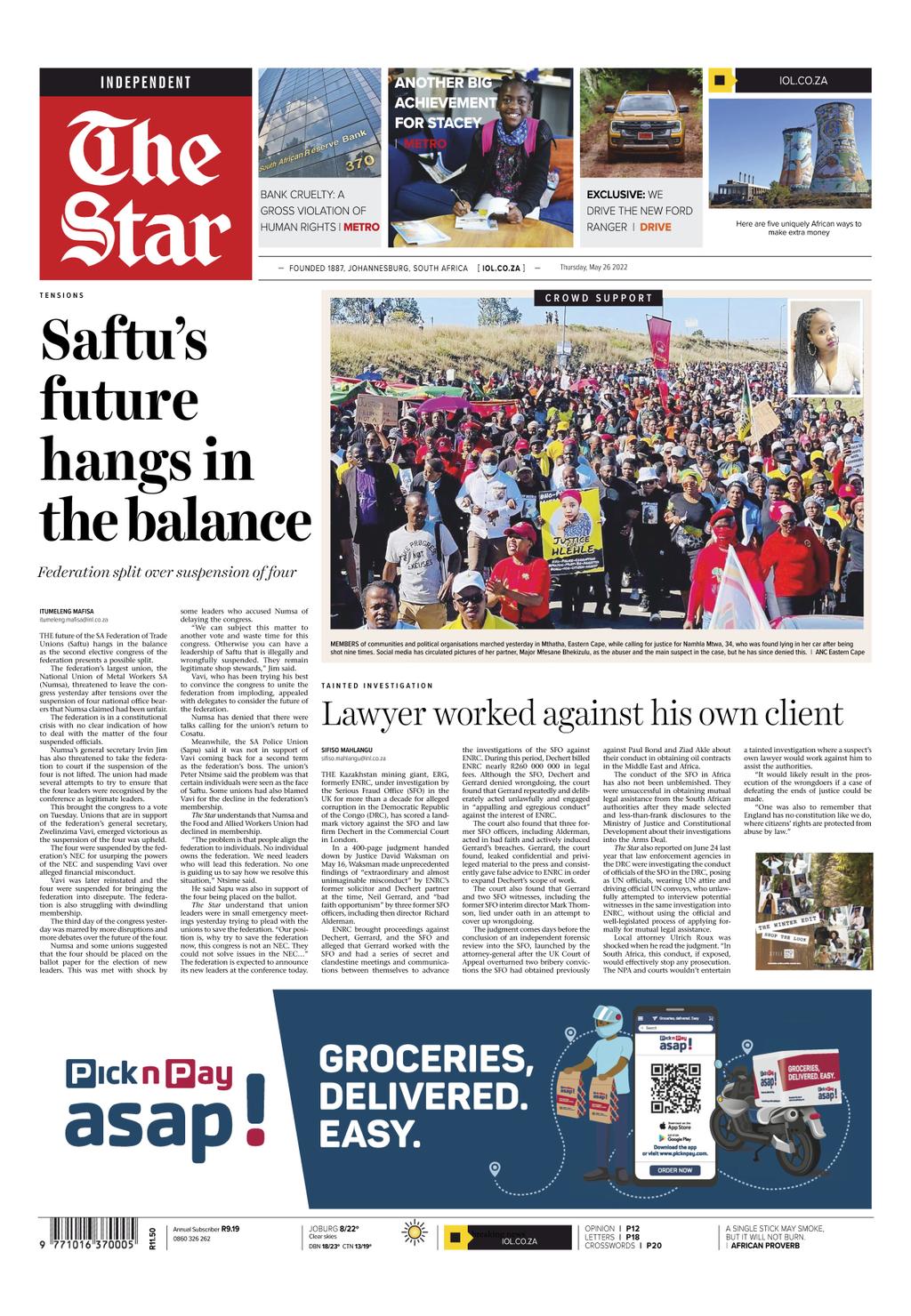**Independent Online Newspaper Screenshot: Analysis**

The image is a screenshot capturing a segment of an online newspaper article. At the top left corner, the publication name "Independent" is prominently displayed in a black bar, signifying the source. Directly below this, in a red box with an old English font, is the title "The Star."

The article title, “SAF2's future hangs in the balance: Federation split over suspension of four,” is positioned beneath the publication name, indicating the main topic of interest. To the right of this title is a photograph depicting a large gathering of people who appear to be either protesting or assembled together for a significant event. The exact nature of the gathering is unclear without additional context.

Beneath the photo is a segment that likely contains a description or caption, although the text is too small to discern clearly. Following this, there is another header stating, “Lawyer worked against his own client,” suggesting another noteworthy article or segment within the publication.

The central portion of the image is primarily filled with the text of the article or news story, providing in-depth coverage of the aforementioned topics. At the bottom of the screenshot, there is an advertisement for “Pick n Pay ASAP,” a service that offers convenient grocery delivery, emphasizing ease and efficiency.